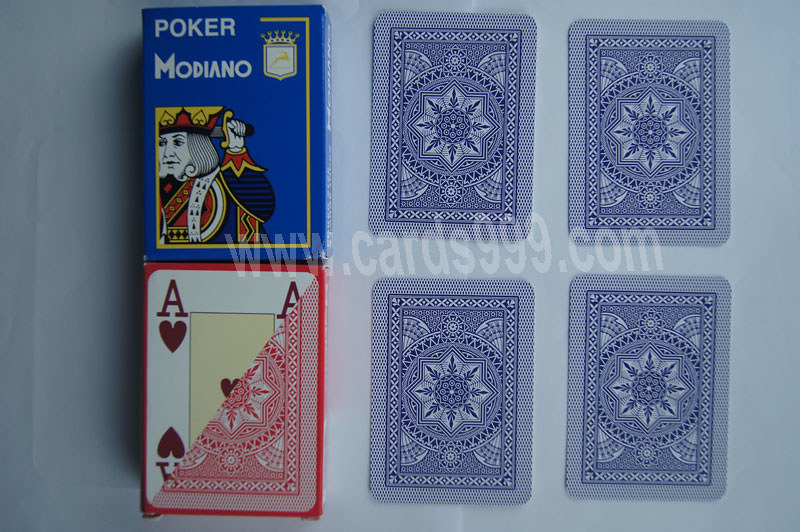In this photograph, playing cards are arranged on a clean, white surface. On the left side of the image, two paper packages of cards are stacked, with one atop the other. The top package is blue, showcasing the text "Poker Modiano" in white font, along with an image of what appears to be the King of Spades in the bottom left corner. Beneath it, a red package features a playing card design cut diagonally, revealing the face of the Ace of Hearts on the top half and the card's red decorated background on the bottom half. 

Additionally, four cards are spread out beside the packages, aligned in two rows of two. These cards display their blue and white patterned backs consistent with a traditional card design. Prominently in the middle of the photograph, a watermark reads "www.cards999.com," indicating the source of the image.